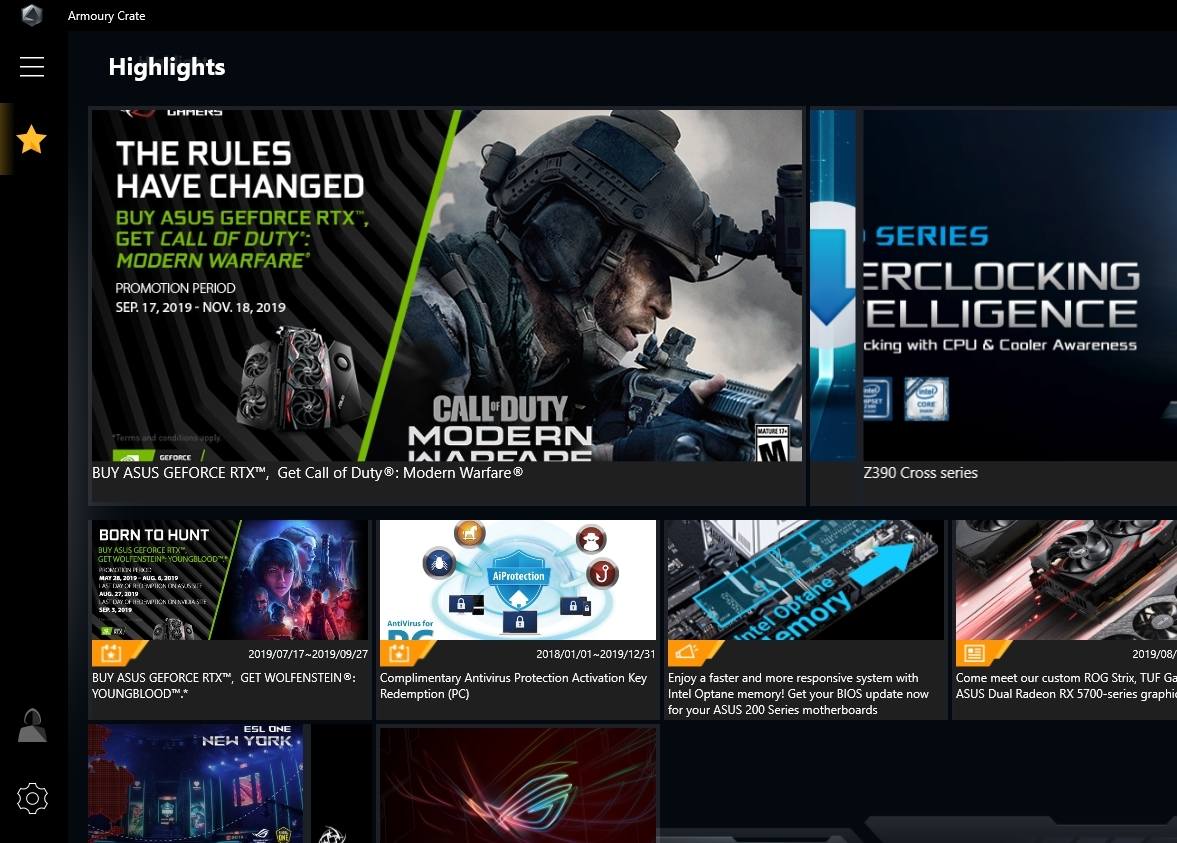An advertisement features an intricate and visually packed display promoting several gaming and PC accessories along with game promotions and offers. 

At the center of the image, a Double S logo is shown prominently next to labels like "Armory Crate" and "Hammergun Manual." Surrounding these, various highlights are noted, including a striking image of a "Yellow Star." Adjacent to this is a promotional picture captioned "The rules have changed" by SSG4STARTX promoting Call of Duty: Modern Warfare, with the offer valid from September 17th, 2019 to November 18th, 2019.

In the background, three "Ghost Cards" are subtly showcased, adding a mystic allure. Complementing these elements, there's a visual of a helmeted soldier holding a rifle, labeled "Call of Duty: Modern Warfare, Matreya."

Moving to the right, a segment titled "Unlocking Intelligence with CPU and Color Awareness" highlights the C390 Crosshair series. On the far left, another promotional image labeled "Born to Hunt" by ACSG4STARTX offers Wolfenstein: Youngblood, featuring exciting, intense graphics.

Additional features include an informative section with a graphic titled "AI Protection," showing a Blue Shield, Yellow Circle, Blue Circle, and Red Circle, highlighting Complimentary Anti-Virus Protection and Activation. There's also a "Cave Redemption PC" feature promising faster and more responsive system performance with Intel Optane Memory. Furthermore, "Biosubject" is available for the ACES 200 Series, promoting the imminent launch of Modern Warfare.

At the very bottom, an invitation to meet their customer on "G-Streak" is extended, cautioning ACES users against reading an article with ACES 200 Series graphics. Finally, a notice about the ESL1 New York event is on a blue background, featuring a mysterious red square with a grey element.

The entire composition is a blend of vibrant colors and captivating visuals, designed to attract and inform gaming and tech enthusiasts.